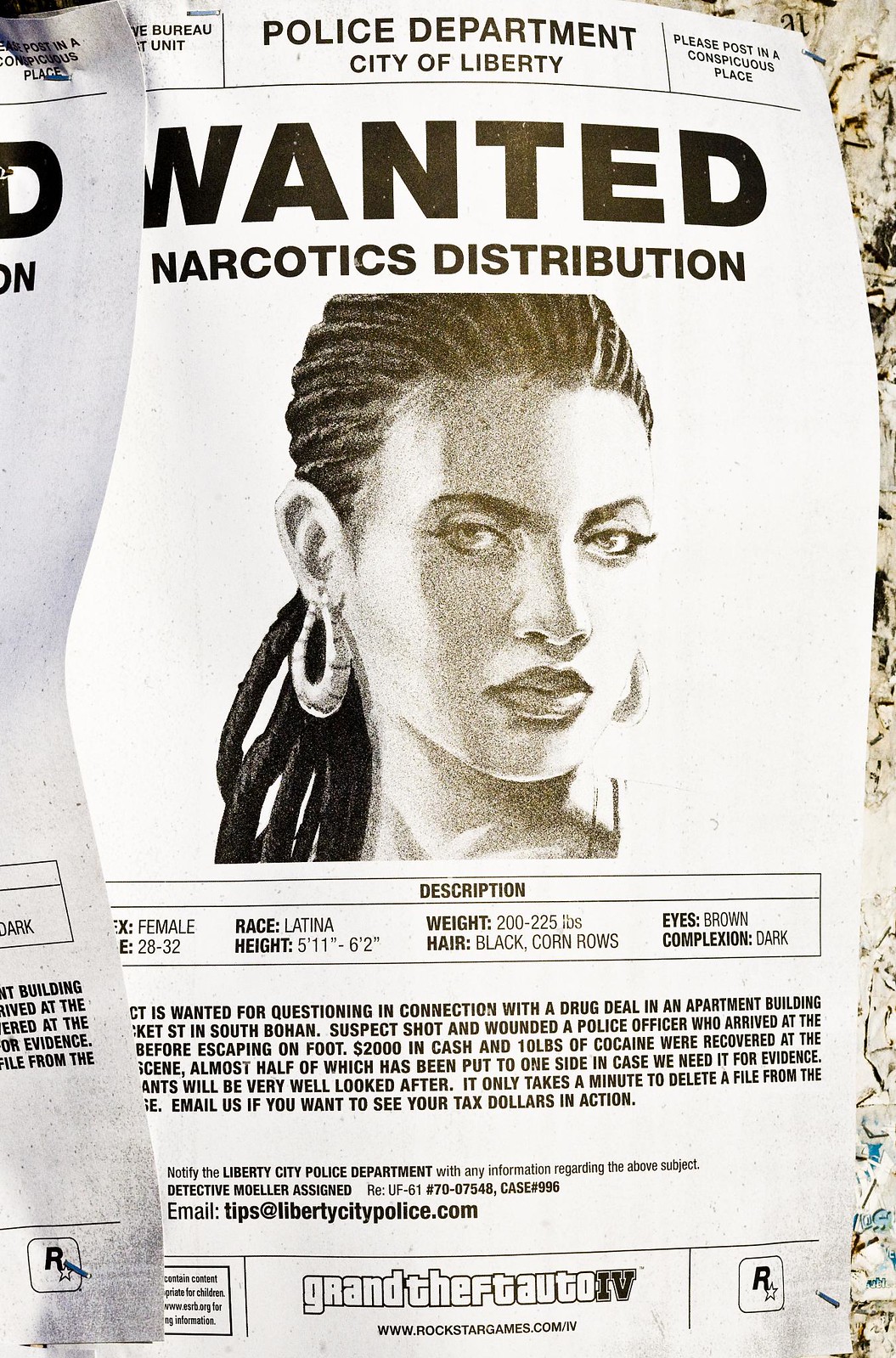The image depicts a black and white artist's drawing styled as a wanted poster, promoting a Grand Theft Auto video game. At the top, "Police Department, City of Liberty" is prominently displayed, followed by "Wanted" and "Narcotics Distribution" in large, bold letters. Below, there is a detailed illustration of a woman with braided cornrows pulled back, wearing large hoop earrings. She is facing forward with no expression. Further down, a table provides a detailed description: Latina, 5'1", 200 pounds, black cornrowed hair, brown eyes, and dark complexion. The bottom of the poster features the Grand Theft Auto logo and URL for RockstarGames.com, along with the Rockstar logo in the lower right corner, indicating the game's rating.